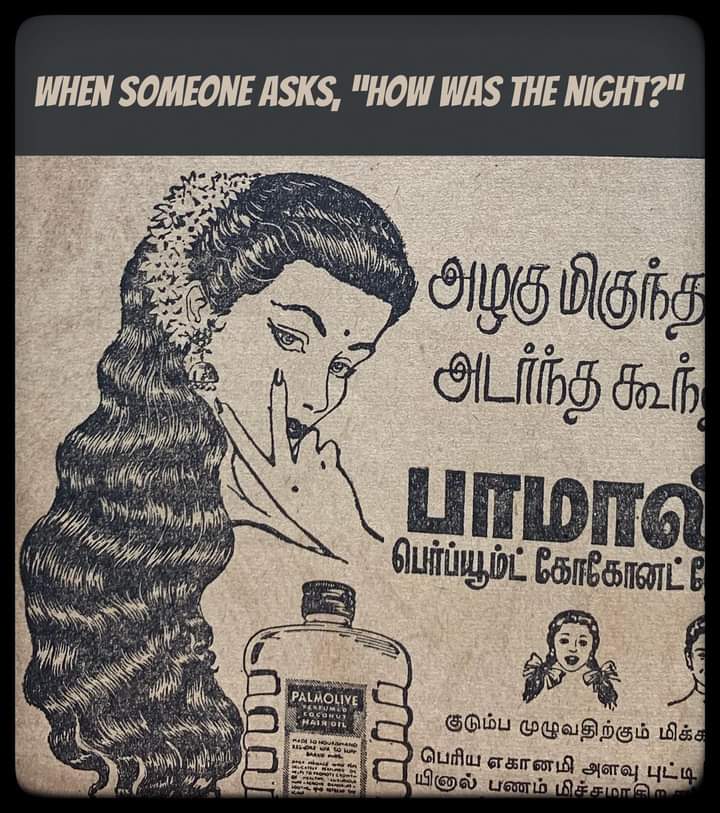This image depicts a vintage advertisement featuring a prominent black banner at the top with white text that reads, "When someone asks how was the night." The bottom part of the ad has an off-white background accented with intricate designs and additional text in black, written in an unfamiliar script that resembles Arabic.

To the left of the ad, there is an illustration of a woman with long, dark hair styled with a wreath of flowers. Her eyes are distinctly almond-shaped, giving an Asian appearance, and she wears elegant earrings. The woman has full lips, meticulously maintained eyebrows, and a bindi—a decorative dot—on her forehead. She strikes a pose with her two fingers touching her cheek, almost in a peace sign gesture.

To the right and towards the bottom of the ad, there is an illustration of a girl with pigtails adorned with bows. At the very bottom center, a jug labeled "Palmolive Perfumed Coconut Main Oil" prominently stands out, making it clear that this is the advertised product. The ad's sepia-toned palette, along with its detailed illustrations and script, evoke an old-time feel reminiscent of advertisements once found in newspapers or magazines.